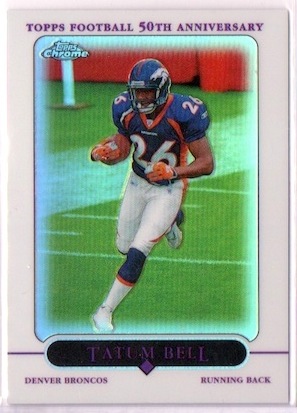This image features a Topps Chrome football trading card commemorating the Topps Football 50th Anniversary. At the top of the card, "Topps Football 50th Anniversary" is prominently displayed in a purplish font. The card showcases a Denver Broncos running back, Tatum Bell, captured mid-action on a green football field, with faint white yard lines visible. Tatum Bell is wearing the team's blue and orange jersey with the number 26 on his chest and shoulders, paired with white pants, blue knee guards, an orange stripe, and white socks and shoes. The player is seen holding the football in his right arm. The card's background includes red barriers likely representing stadium stands. The bottom of the card features "Denver Broncos" and "Running Back" also in the purplish font. Tatum Bell's name is printed in a dark, somewhat challenging-to-read blue or black font against a black background with a diamond graphic at the center bottom. The card has a white border with rounded corners, adding to its classic trading card aesthetic.